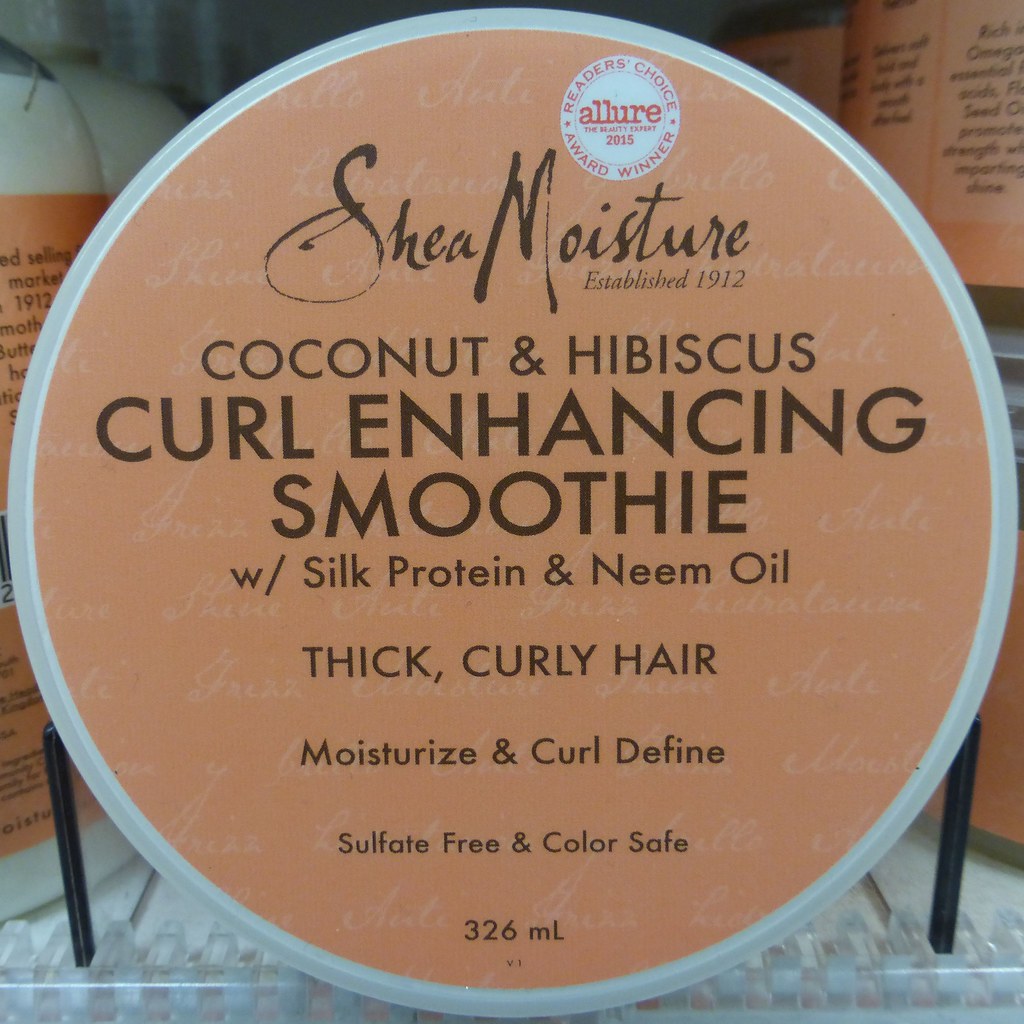The image depicts a close-up of a round, silver-lidded jar, with a light coral or peach-colored label. The label is densely covered with text, primarily in dark brown writing. At the top, "Shea Moisture" is written in cursive, followed by "Coconut & Hibiscus, Curl Enhancing Smoothie with Silk Protein & Neem Oil." Additional details include "Thick Curly Hair," "Moisturize & Curl Define," "Sulfate-Free," and "Color Safe." The label also indicates the jar’s size as 326 milliliters. In the background of the label, white text appears to repeat, possibly saying "Allure 2015 Reader's Choice Award Winner" or similar accolades.